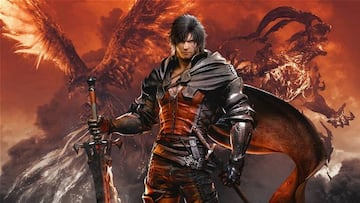In this image, we have an intricately detailed character that appears to be from a video game or a fantasy-themed creation, possibly inspired by Japanese manga or medieval comics. The central figure is a man with long black hair, clad in a dramatic, visually striking outfit. He wears a metallic black cape and a tight-fitting leather attire predominantly black with a distinguishing orange design running down the center and complemented by a metallic reddish breastplate. His arms are adorned with substantial armor, one sleeve is metallic, leading to a metal-gloved hand. In his left hand, he holds a sword pointed downwards, though some descriptions suggest it could be a gun.

The background is dominated by intense hues of orange and red, evoking a fiery, apocalyptic setting. Smoke and a red sky enhance the scene's dramatic effect. Behind the character, an enormous, fiery phoenix can be seen soaring, itself seeming ablaze. To the upper right, a looming demonic figure enveloped in flames and sporting horns adds to the scene's epic and chaotic atmosphere. Additional mechanical devices and elements are scattered around, hinting at advanced technology or magical artifacts within this vividly illustrated world.